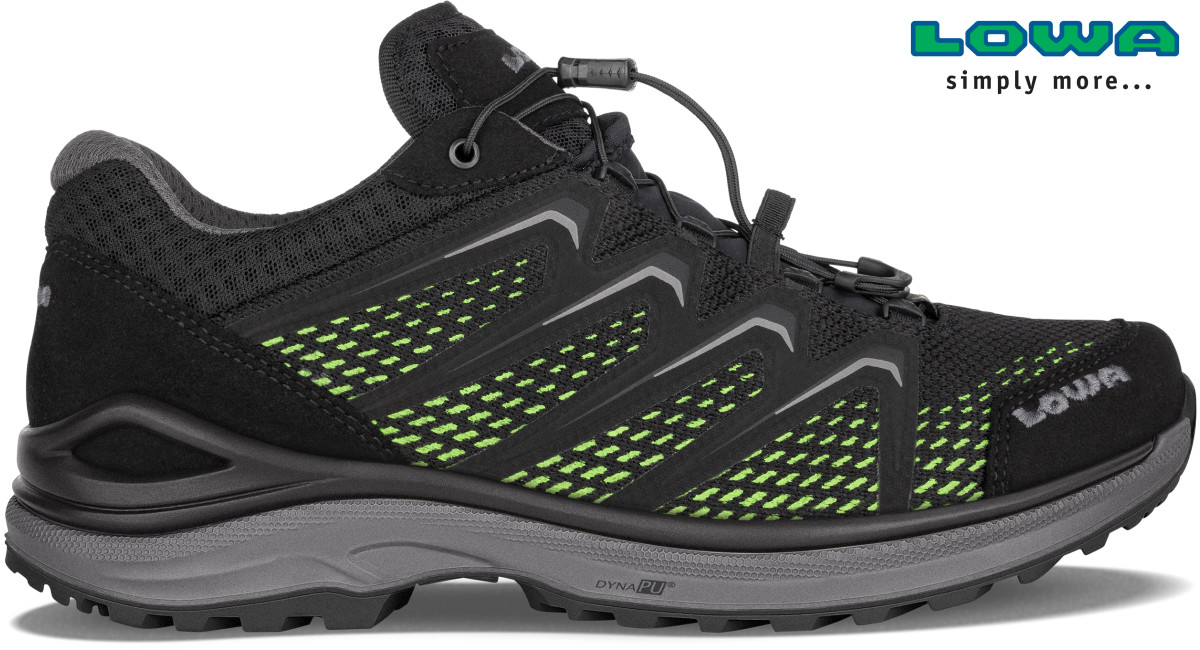The image portrays a detailed side view of a black trail running shoe from the brand LOWA. The shoe features a predominantly black mesh exterior with neon green speckles adding a pop of color. Its sole showcases a distinct contrast: the upper sole is light gray, while the bottom tread remains black, providing excellent grip. A unique feature of the shoe is its Dynapu (D-Y-N-A-P-U) technology embedded in the sole, ensuring enhanced durability and comfort. The shoe is fastened with a black string lace system, designed for easy pull-and-secure functionality. Inside, it appears cushioned with foam for added comfort. The brand's name, LOWA (L-O-W-A), is prominently displayed on the heel in grey text and again on the tongue of the shoe. The shoe is set against a white background, casting a subtle gray shadow. In the top right corner of the image, green text with a blue outline reads “LOWA” with the tagline “simply more...”. This comprehensive image showcases the blend of functionality and style in a trail running shoe.